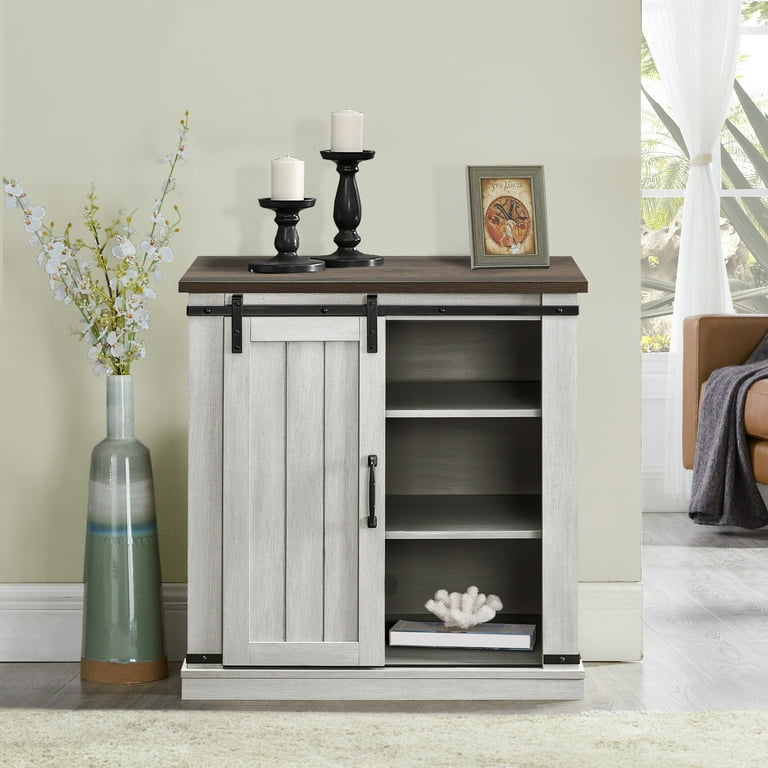This detailed photographic image captures an indoor room setting, potentially a blend of bedroom and living room elements. The focal point is a white wooden cabinet with an open door revealing three greyish shelves inside. The bottom shelf holds white stones arranged in a bouquet fashion. Atop the cabinet is a dark brown countertop featuring two brown candle holders with white candles, the right candle holder being taller than the left. Next to the candles sits a framed print of a person inside a circle, enclosed in a green frame. 

To the left of the cabinet is a tall cylinder-like vase, adorned with bands of grey and blue, filled with a multitude of flowering plants with white blossoms. The wall behind the cabinet is light grey, and this section transitions to reveal a partial view of another room. In this adjacent room, there is a brown sofa draped with a grey or purple blanket, positioned next to a window flanked by a curtain. The floor in the foreground is marble, accentuating the overall clean and minimalist aesthetic of the room.